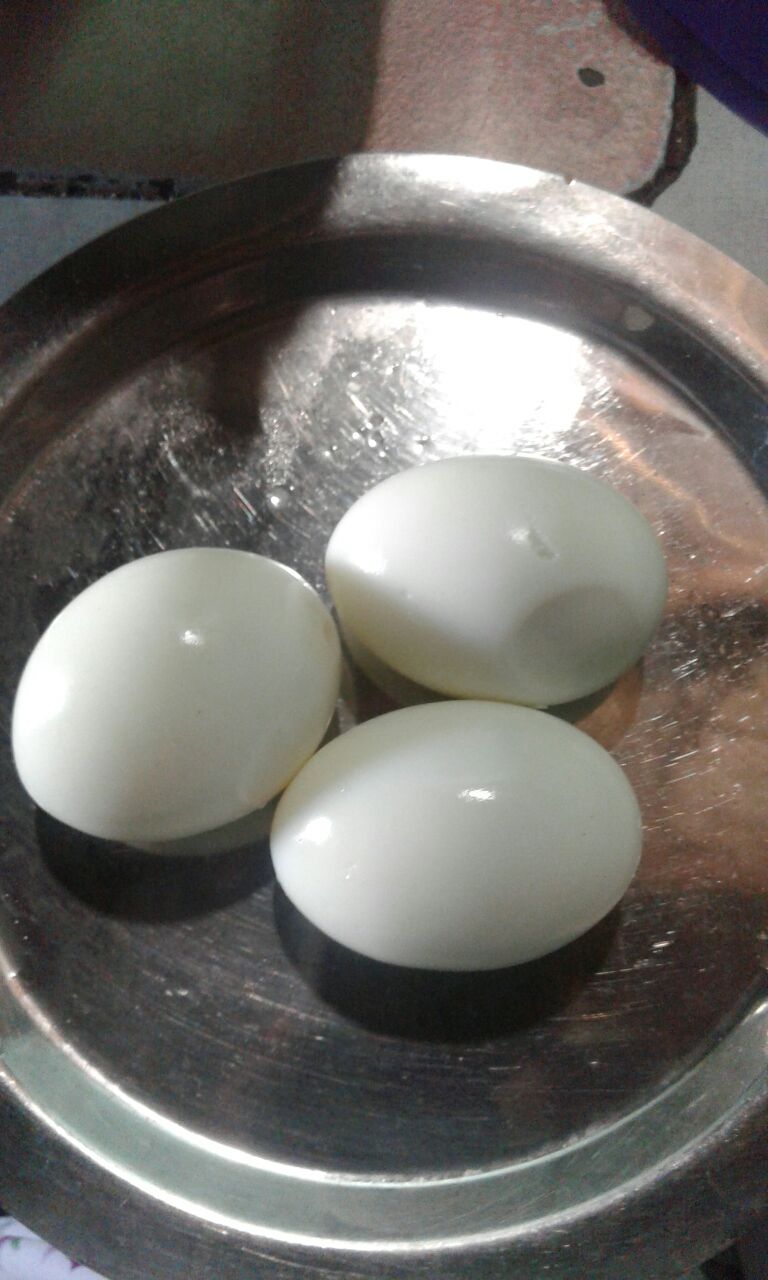This is a vertically oriented, color photograph showcasing a round, silver metal bowl positioned on a gray or brownish table. Inside the bowl, three white, peeled hard-boiled eggs are arranged in a triangular formation, with one egg lying horizontally at the bottom and the other two positioned slightly diagonally above it. The eggs exhibit patches of a jelly-like substance or reflective spots indicating light reflection. The metal surface of the bowl catches the light, creating a striking silvery glare and contributing to a slight blurriness at the upper portion due to the brightness. Beyond the bowl, there appears to be a brownish tray with shadowing, and in the background, a black Sharpie-drawn rectangle can be discerned on the table. Additionally, a shadow is noticeable in the right corner of the image.